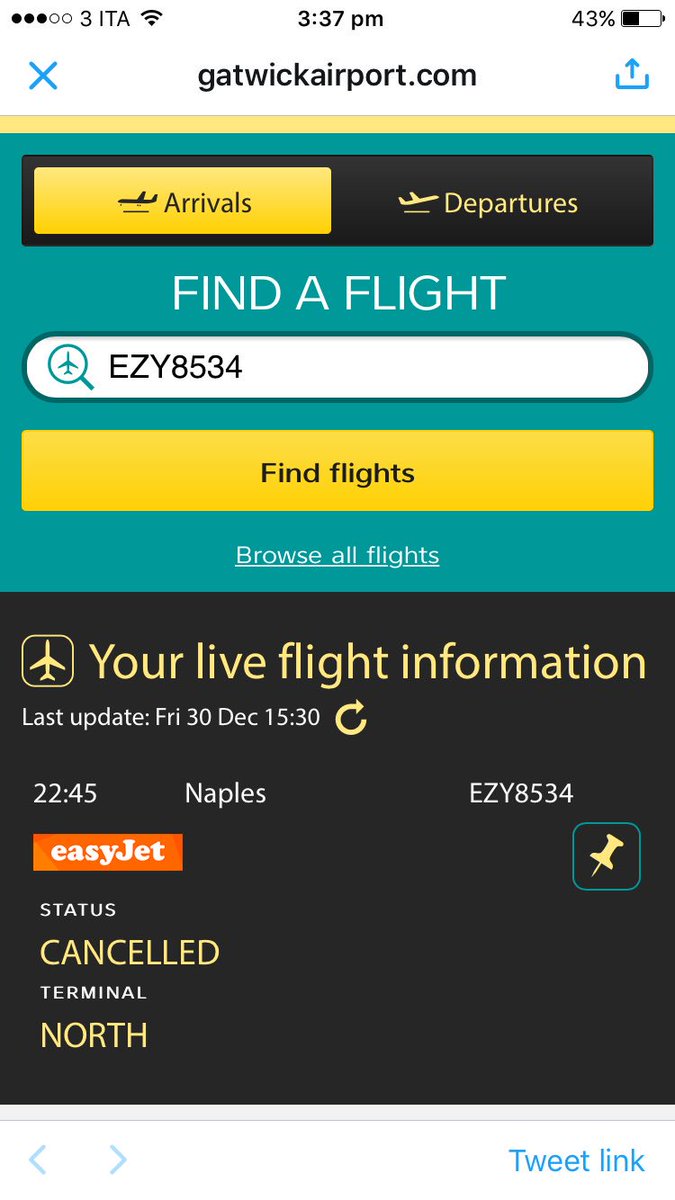Sure, here is a cleaned-up and detailed description of the image:

---

The image is a screenshot of a mobile phone displaying a webpage from Gatwick Airport. At the top of the screen, the status bar shows "3 ITA" indicating the carrier, an internet connection symbol, a battery level of 43%, and the current time as 3:37 PM, all written in black.

The webpage itself has several sections. At the very top, there is a URL bar showing "gatwickairport.com", with options to type in and download content.

Below that are two tabs: "Arrivals" and "Departures." The "Arrivals" tab is selected, highlighted with a 'Go' button next to it. The "Departures" tab is in black, and within this section, there is a text field for entering flight numbers, along with a "Find a flight" button.

Beneath these tabs, the background color changes to green with blue and light blue text options. There is a clickable link labeled "Browse all flights."

Further down the page is an icon of an airplane accompanied by information stating "Your live flight information, last update: Friday, 30th of December, 15:30" (or 3:30 PM in military time). This section also includes an option to refresh the information.

Highlighted next in the flight details, it lists:
- Flight Number: 2245
- Destination: Naples
- Airline: EasyJet

Next to this, there is a pushpin icon indicating that users can interact with it. The status of this flight is marked as "Cancelled" with a note that it was supposed to depart from Terminal North, followed by a red notification stating, "Cancelled."

---

This should provide a clear and detailed overview of the screenshot described using a clean and structured format.